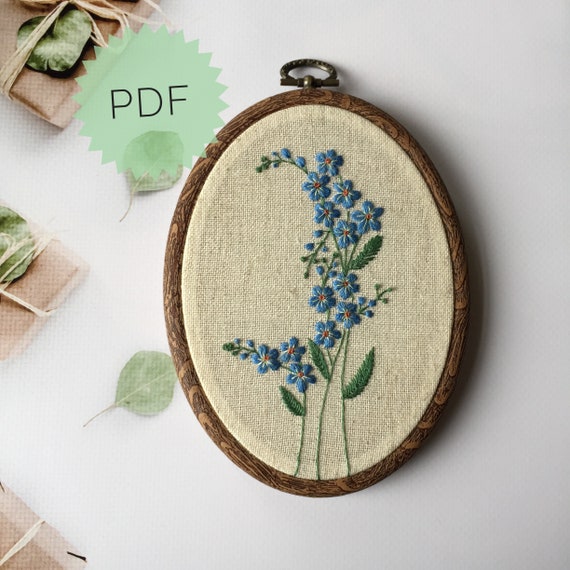The photograph is a horizontally aligned rectangular image featuring a round embroidery artwork positioned centrally and slightly to the right. The piece is encased in a brown and tan circular wooden frame with an intricate pattern of grays and tans on the outer edges. At the heart of the embroidery, a beige cotton canvas is meticulously stretched and trimmed. The embroidery itself presents a delicate design of blue flowers with green stems and leaves, some of which bud and arc gracefully to the left at both the top and bottom. The flower centers are highlighted with an orange-brown hue, adding contrast and vibrancy.

At the top of the wooden frame is a yellowish metal, possibly bronze or brass, designed for hanging. This metal fixture includes a bead-like element and a bar spanning approximately one centimeter on either side, culminating in a loop for mounting.

The image’s background is a gradient of very light blue, transitioning to a darker blue on the right side, where the shadow of the wooden frame is visible. In the top left corner, a jagged, semi-opaque, light green starburst with roughly 30 points displays the capitalized black letters "PDF." Further embellishing the starburst, there is a near-circular leaf with pointed ends aligned diagonally, repeated about 6 centimeters below.

To the left side of the image, multiple flat, square brown packages are visible, bound with natural fiber twine in a crisscross pattern. Scattered green leaves are interspersed among these packages, adding a touch of nature to the composition. This detailed setting captures an intricate mix of craftsmanship, natural elements, and organization in a visually engaging arrangement.